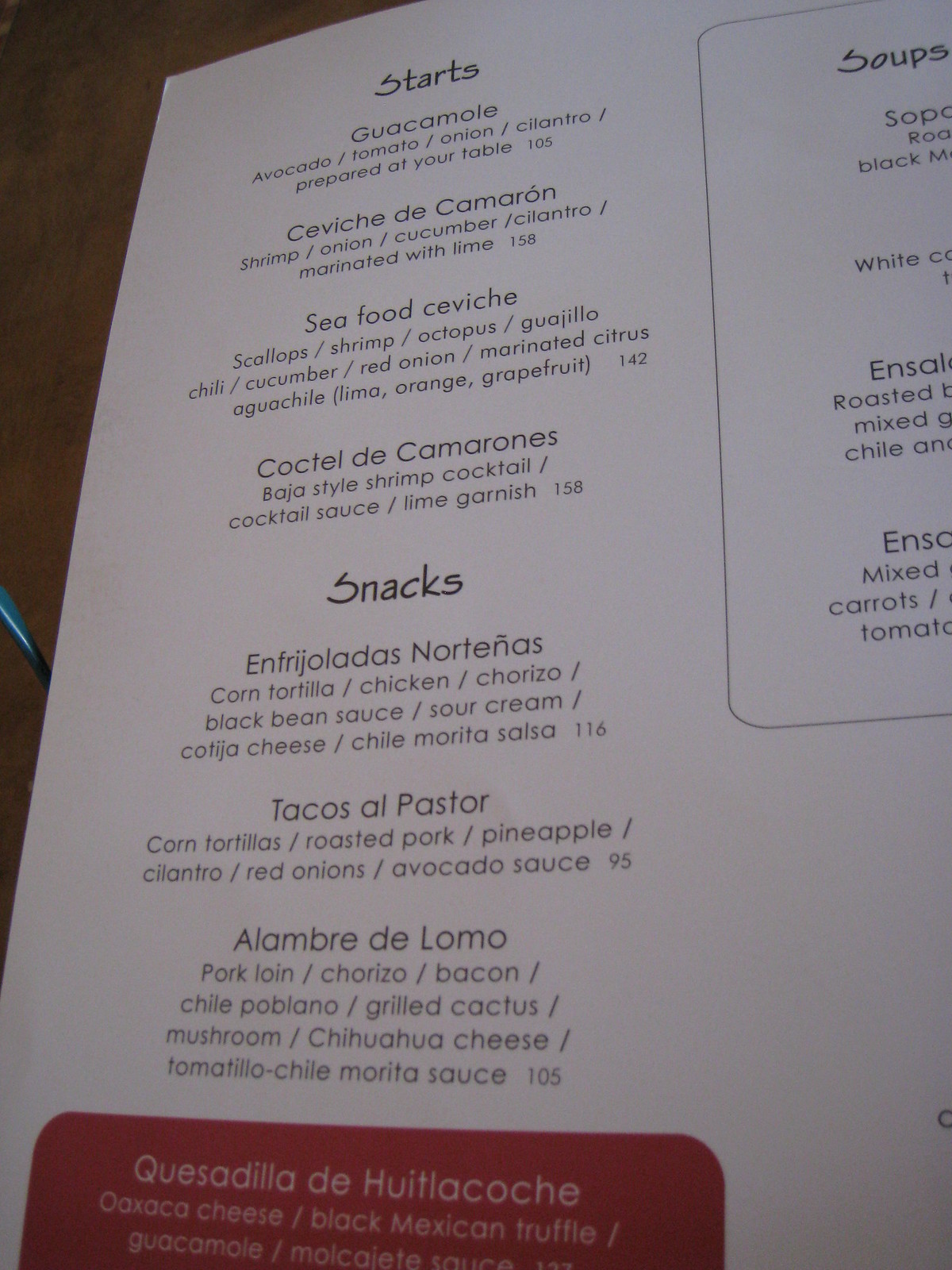This image is a detailed color photograph of a portion of a menu from what appears to be a Mexican restaurant. The menu is printed on white paper and is laid out on a wooden table. The text is primarily in black font, providing a stark contrast against the white background.

At the top of the visible portion of the menu, in bold letters, it says "Starts," under which are listed various appetizers, including guacamole, ceviche de Camarón, seafood ceviche, and cocktail de Camarones, each with detailed descriptions of the ingredients.

Below the "Starts" section is another bold heading that says "Snacks." This section includes a variety of snack options with detailed descriptions as well. Some of the listed items are tacos El Pastor, Alhambra de Lomo, and frijolitos norteños.

At the bottom of the snack section, there is a small red square with white text that highlights a dish called quesadilla de huitlacoche, accompanied by a description of the dish’s ingredients.

On the right side of the menu, part of the word "Soups" is visible, indicating that various soup options are listed below, although this section is partially cut off in the photograph.